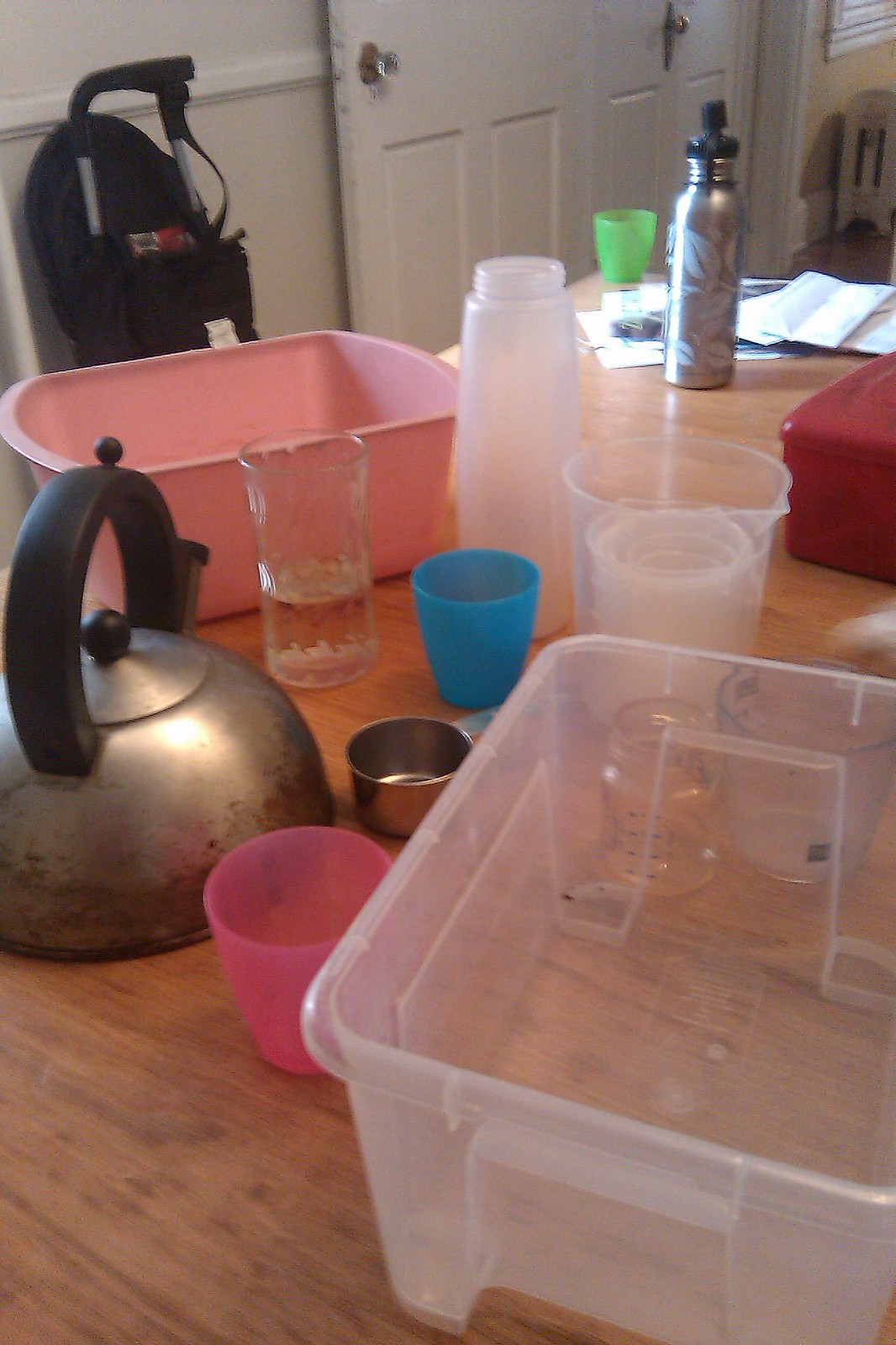Here is a cleaned-up and more detailed caption for the image:

---

A wooden table is covered with various items, including four cups: a medium pink cup, a small silver cup placed above it, a medium blue cup to the left, and a tall glass filled with water to the leftmost side. To the right of the glass is a measuring cup, and aligned with the silver cup on the left is a tea kettle. Further to the right of the tea kettle is a clear Tupperware container. Next to the tall glass is another pink Tupperware on the right, and adjacent to that is a bottle missing its top. On the top right corner of the table, there is a thermos or a container used to keep drinks cool. Slightly upwards and to the left of the thermos, there is a cream-colored cup. The table is also scattered with papers. At the far left end of the table, there appears to be a black bag or backpack. The setting includes wooden doors and a wooden floor.

---